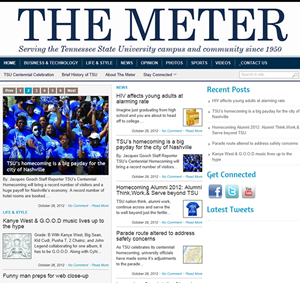This image features a newspaper-style page titled "The Meter" in bold at the top. Below the title, it reads, "Serving the Tennessee State University campus and community since 1950." Centrally placed is a picture depicting university learners engaged in campus activities. 

The page contains various articles, including a blog about the alarming rates at which HIV affects young adults. It also highlights significant events such as TSU's homecoming, which reportedly provides a substantial financial boost for the city of Nashville, and discusses the involvement and achievements of 2012 alumni, encouraging them to continue working and serving beyond TSU. There is mention of parade routes being adjusted to address safety concerns. 

Another article reviews Kanye West's music, noting that it lives up to the hype, and there is an assortment of recent posts listed on the side of the page. The page also features social media icons for Facebook, Twitter, and YouTube, albeit in older designs, indicating a connection to these platforms for further engagement.